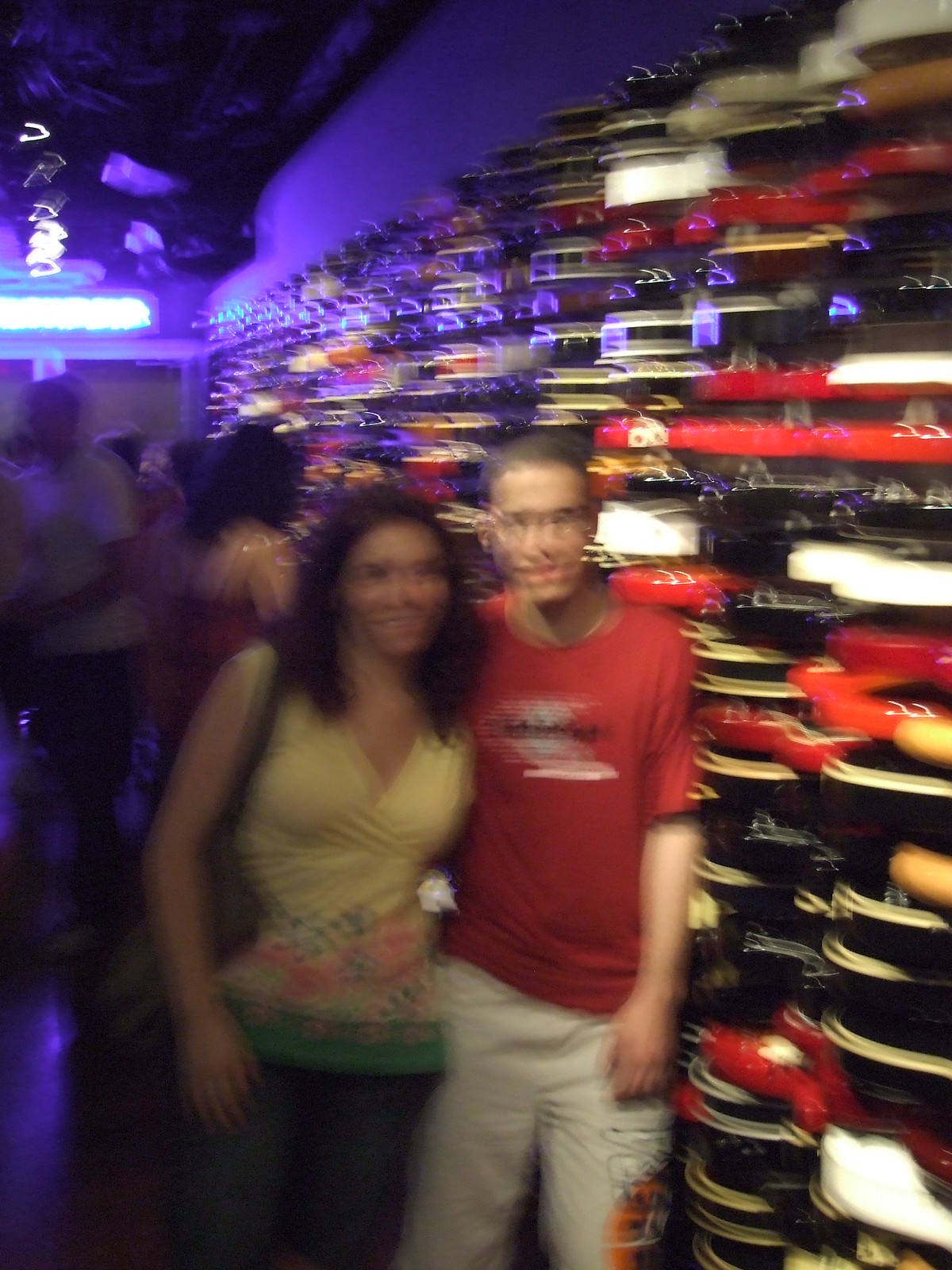A slightly out-of-focus image capturing a young couple posing and smiling under ambient purple mood lighting. The man, sporting short hair, is dressed in white trousers and a red t-shirt, while the woman beside him, with long dark hair, wears a sleeveless green and yellow top featuring a green band at the bottom. This scene takes place in a busy setting, with indistinct men and women milling around in the blurred background. They stand near a tall shelf, approximately 10 feet high, filled with colorful but indiscernible items. The overall backdrop is vibrant, despite the image's lack of clarity, and the couple's expressions convey happiness within a lively, bustling environment.